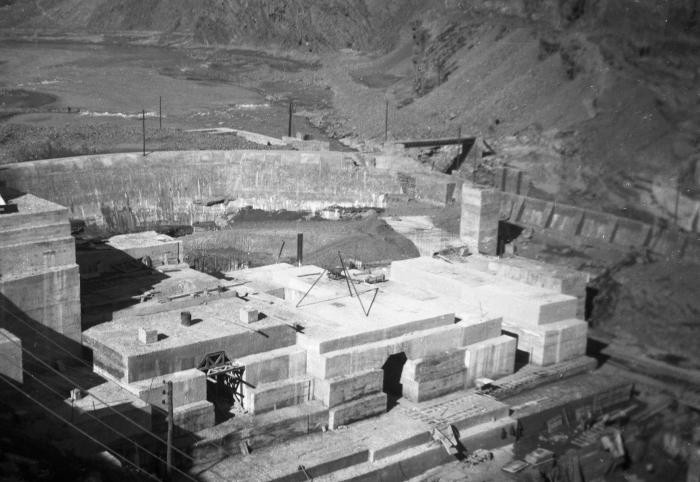The black-and-white image presents an excavation site with a distinct contrast of dirt and stone elements, possibly depicting an archaeological dig, a construction site, or a potential bomb shelter. The scene features a substantial amount of concrete and large stones resembling an ancient, heavily fortified structure or an emerging foundation. Visible within the site are arched stone or limestone structures, which might include steps and a platform, scattered amidst what looks like a clearing or a crater-like formation. Entrances and openings suggest an intricate architecture possibly belonging to a vault, a government facility, or similar. No individuals are present in the image, adding an eerie stillness to the location. Machinery and vehicles are stationed at the forefront, while the periphery is enclosed by walls, railings, and barriers. The backdrop features a non-lush landscape with surrounding hills and a potential gravity dam, devoid of water. Sparse poles, likely for utility purposes, are also seen, emphasizing the site's barren, utilitarian nature.